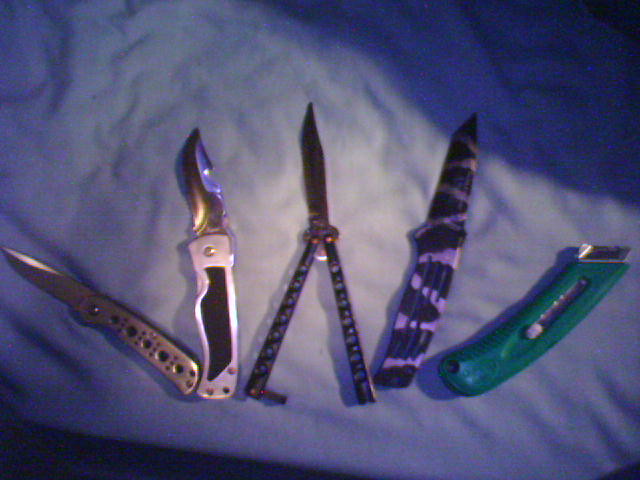The image depicts a group of five knives arranged on a blue, wrinkled blanket that could be draped over a bed. The photograph captures the scene with a central light source, creating a bright spotlight in the middle and casting shadows towards the upper right and lower left corners. 

Starting from the left, the first knife is a fully silver pocket knife featuring multiple holes in its handle and a foldable blade. Next to it is a knife with a white handle accented with black, likely another pocket knife with a distinctive design feature of a silver blade and a bottle opener. The third item is a butterfly knife that stands out with its striking purple handles adorned with either a leopard or giraffe print that extends onto its blade. Moving further right, the fourth knife, often described as tactical, has a black and pink handle with claw mark-like patterns on it. Lastly, on the far right, there is a simple green box cutter, noted for its retractable blade that is currently extended about a quarter-inch.

The entire setup suggests a display under low light conditions, highlighting the varying sizes, colors, and designs of each knife against the soft, undulating cloth background.